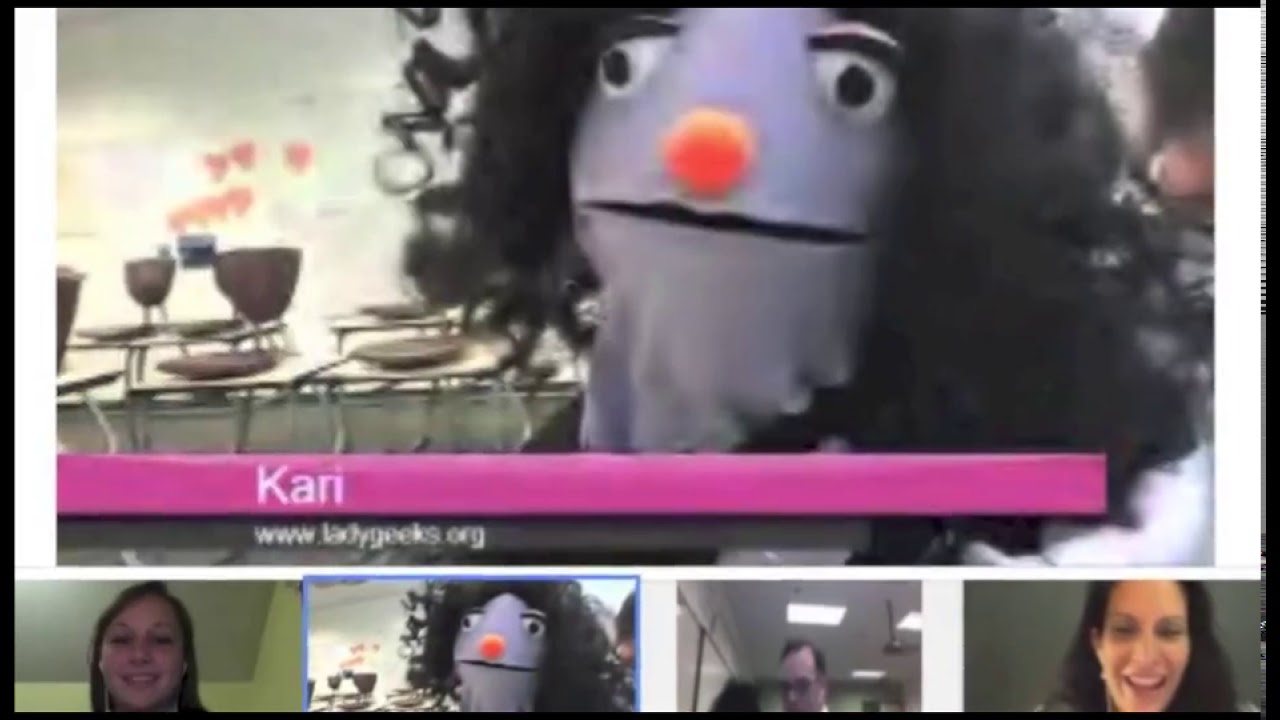This is a detailed description of a wide rectangular screenshot capturing a video chat, framed by a thin black border. Dominating the top three-quarters of the image is a large rectangular frame featuring a purple puppet with an orange nose and long, black curly hair. Behind the puppet, identified by the text "Carrie" on a pink strip at the bottom of her screen, is a classroom setup with brown desks and chairs, along with a wall adorned with posters. Below the main frame are four smaller frames in a horizontal line. The first frame shows a woman with brown hair against a beige background. The second frame is a smaller version of the image of Carrie, the purple puppet. The third frame captures a man under a ceiling, while the fourth frame features another smiling woman with brown hair. The scene resembles a Zoom call or Skype meeting, with the main participant being the puppet named Carrie.